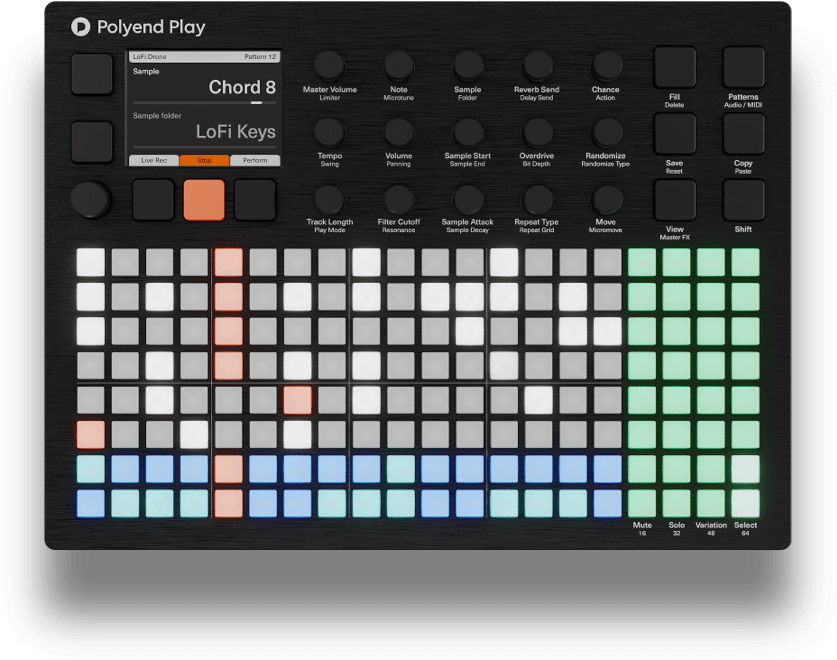This image depicts a sophisticated piece of black recording and sound equipment featuring an array of buttons, knobs, and a vibrant grid interface. In the top left corner, there's a screen displaying various commands: "Lo-Fi Pattern 12," "Sample Chord 8," "Sample Folder Lo-Fi Keys," "Live Recording," "Stop," and "Perform." Accompanied by the logo—a small 'P' and branding "Polyend Play"—this technology piece is equipped with numerous controls including "Master Volume," "Note," "Sample Folder," "Reverb Send," "Chance Action," "Randomize Type," "Move," "Repeat Type," "Overdrive," "Sample Start," "Sample Attack," "Filter Cutoff," "Volume," "Tempo," "Track Length," "Fill," "Patterns," "Save," "Copy," "View," and "Shift." Notably, the bottom portion of the device features an organized grid of squares in various colors, such as white, blue, red, green, and peach. Although some keys look like piano keys, the device primarily consists of round and square buttons designed for intricate sound and recording manipulation. This equipment appears to be tailored for creating and modifying musical recordings with an intuitive and colorful interface.